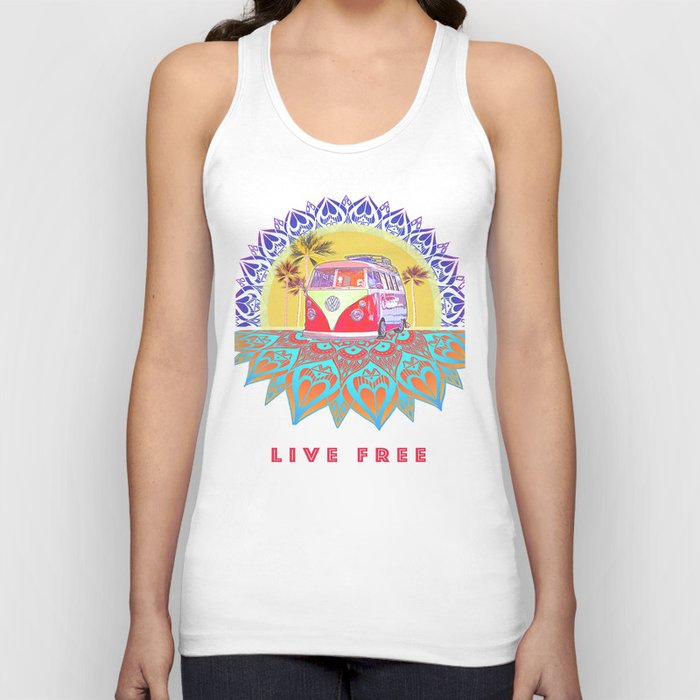In this image, we see the bottom half of a young woman captured from below her chin to around her hips, against a white background. She is wearing a white tank top that exposes her collarbone and arms, which hang straight down by her sides. The tank top features a vibrant, hippie-inspired graphic centered around an illustration of a classic Volkswagen bus, complete with round headlights, a luggage rack on top, and the VW logo prominently displayed in the V section of the design. Surrounding the bus are palm trees and intricate, psychedelic patterns in blue, red, and orange hues. The entire graphic is framed by blue ornamental decorations and complemented by red and yellow flower-like designs. Below the illustration, bold text with a thick red outline reads, "Live Free." The model is also wearing blue jeans, completing her casual, free-spirited look. The overall color scheme of the graphic includes black, white, red, cream, blue, orange, and green, enhancing the retro, trippy aesthetic of the design.